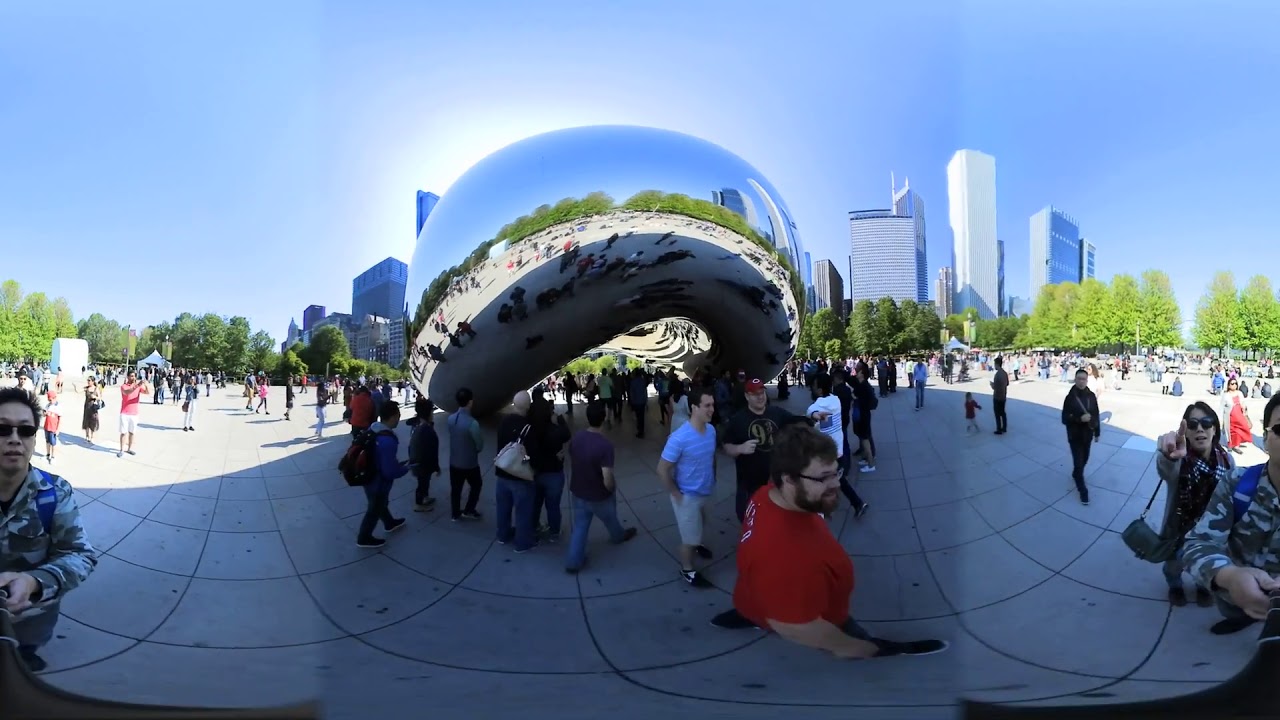This vibrant summer image captures a bustling scene at Chicago's iconic Cloud Gate, commonly known as "The Bean." Positioned centrally, the large, reflective silver sculpture showcases a multitude of pedestrians dressed in warm-weather attire, including shorts and short sleeves, as they mill about on the surrounding paved area. The Bean's smooth surface mirrors the activity around it, displaying reflections of people in various postures: directly in front, a man in a red shirt with glasses looks away, while a man in a blue shirt and khaki shorts, and another in a black shirt with a baseball cap, are nearby. Particularly noticeable is a woman on the right, pointing at the camera, wearing dark sunglasses and carrying a dark purse. 

In the broader panorama, the image's 360-degree view encapsulates the surroundings beautifully. To the right, green trees line the area before towering skyscrapers, all under a vivid, cloudless blue sky. The photographer, identifiable by his camouflage-patterned shirt and sunglasses, appears twice due to the panoramic nature of the shot. The lively, bright day is punctuated by clear shadows cast by the pedestrians and the Bean itself, enhancing the sense of depth and realism in this striking capture of a quintessential Chicago landmark.